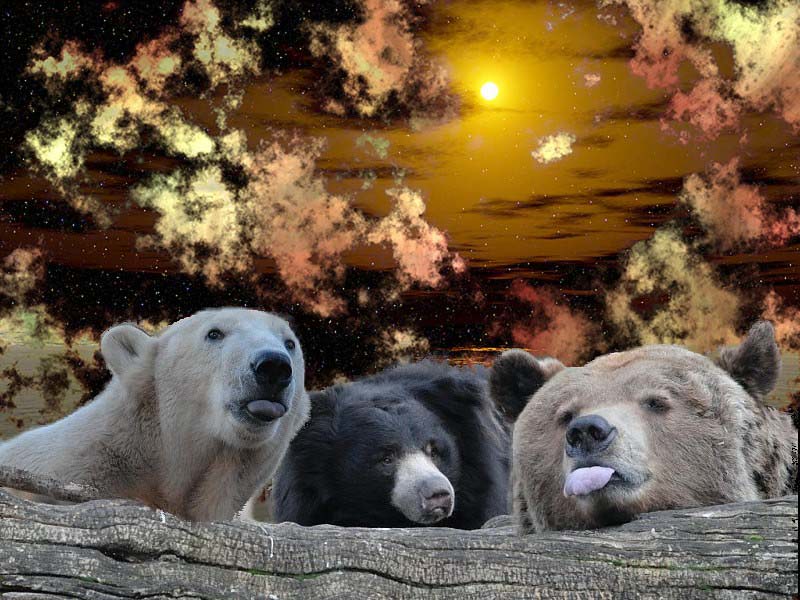The image features a captivating and surreal scene, seemingly AI-created or heavily photoshopped. Central to the composition is an aged, chipped, and warped wooden log. On top of this log rest three distinct bears. On the left, a tan-colored polar bear with a black nose and its tongue playfully sticking out of its snout peers out with both eyes visible. The middle bear is a black bear with a white snout and light-colored nose, presenting a comical, pouting expression as it stares rightward with closed lips. On the right, a brown grizzly bear with ears perked up rests its head on the log, showing off its lighter tan snout and hint of a purple tongue. The backdrop of this intriguing image is a dramatic, golden sunset with bright yellow clouds and interspersed celestial bodies in hues of yellow and pink, adding an otherworldly and intensely contrasted sky. The bears appear to have some artifacting around them, suggesting they were digitally inserted into the vividly contrasting scene of a starry twilight sky.